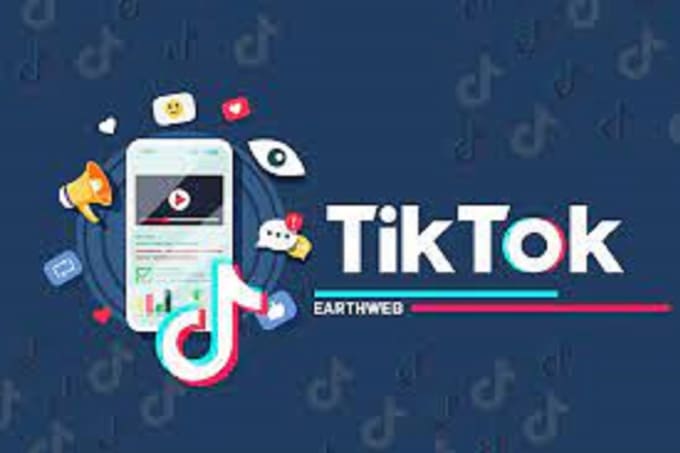The advertisement for TikTok features a predominantly navy blue background, almost square in shape but slightly wider than it is tall. Positioned slightly to the left of the center is a highly detailed cell phone icon showcasing a video with a play button, symbolizing the app's primary function. Surrounding the phone, various vibrant icons and emojis are scattered, including a megaphone, a smiling face, a heart, an eye, a chat bubble with three dots, a red exclamation mark, a larger "T", a thumbs-up like button, and another heart, adding a playful and engaging element to the visual.

Prominently displayed are the words "TikTok" in distinctive font, split into two lines: "T-I-K" on the first line and "T-O-K" on the second. The text is underlined by a bold aqua blue line starting from the first "T" and extending to the "O" in "TOK", followed by another underline in bright pink starting from the "K" in "TIK" and stretching slightly past the final "O" in "TOK", creating a dynamic double underline effect. Below this is the phrase "earth web", also underlined in bold red, adding an additional layer of color and emphasis to the design. This captivating arrangement of elements underscores TikTok's vibrant and dynamic nature, drawing attention to the app’s lively community and interactive features.